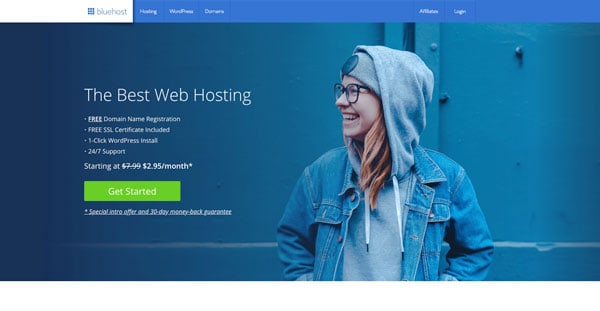The horizontal image appears to be a screenshot from a website, viewable on both computers and smartphones. At the top, the interface includes a white header with a light blue grid, displaying the text "Bluehost" across it. Immediately below is a long, rectangular blue strip featuring a series of clickable options. Positioned to the right side of this strip, additional clickable options include a login button, set against a tealish background.

The main visual focus is a woman standing outside, in front of a wall. She is wearing glasses, a beanie, a hooded jacket with the hood up, and a jean jacket. Her hands are in her pockets, and the image is cropped just below her stomach. 

To the left of the woman, text promotes Bluehost’s web hosting services, highlighting features such as:
- Free domain name registration
- Free SSL certificate
- One-click WordPress installation
- 24/7 support

The promotional text indicates a pricing model with an initial crossed-out rate of $7.99/month, replaced by $2.95/month accompanied by an asterisk. Below this, a green button with white text prompts users to "Get Started." Further details clarify that the reduced price is a special introductory offer with a 30-day money-back guarantee, the latter part underlined for emphasis.